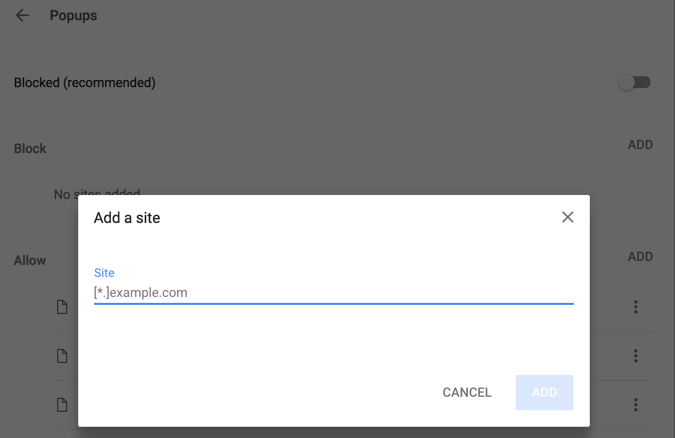The image features a pop-up overlaying a webpage. The pop-up is a white rectangular box. In the top left corner, the word "ADD" is written in black capital letters. To the right of this, in the top right corner, there is a gray "X" icon for closing the pop-up. Beneath the title, the word "SITE" is displayed in blue uppercase letters. Next to "SITE" in black text, within parentheses, there is a star symbol followed by a period and then "example.com".

At the bottom of the pop-up, there are two buttons. The left button is gray with the word "Cancel" in white text. The right button is a light blue box with the word "ADD" in all capital white letters.

The pop-up partially obscures the underlying page, which has a dark gray filter over it. Visible on the main page, albeit dimmed, is a black or gray arrow pointing left. Next to this arrow, the word "Pop-ups" is written in black text. Under this, there is a bit of space followed by the word "Block" in bold black capital letters, with "(recommended)" in parentheses next to it. Below this, in gray text, is the word "Block" again.

Further down and slightly obscured, the word "Add" in capital letters is visible, followed by "No". The words "sites added" can be partially seen, though partially obstructed by the pop-up. Also visible are the word "Allow" and three icons on one side, with the word "Add" in all capital letters and three stacked sets of three circles on the other side.